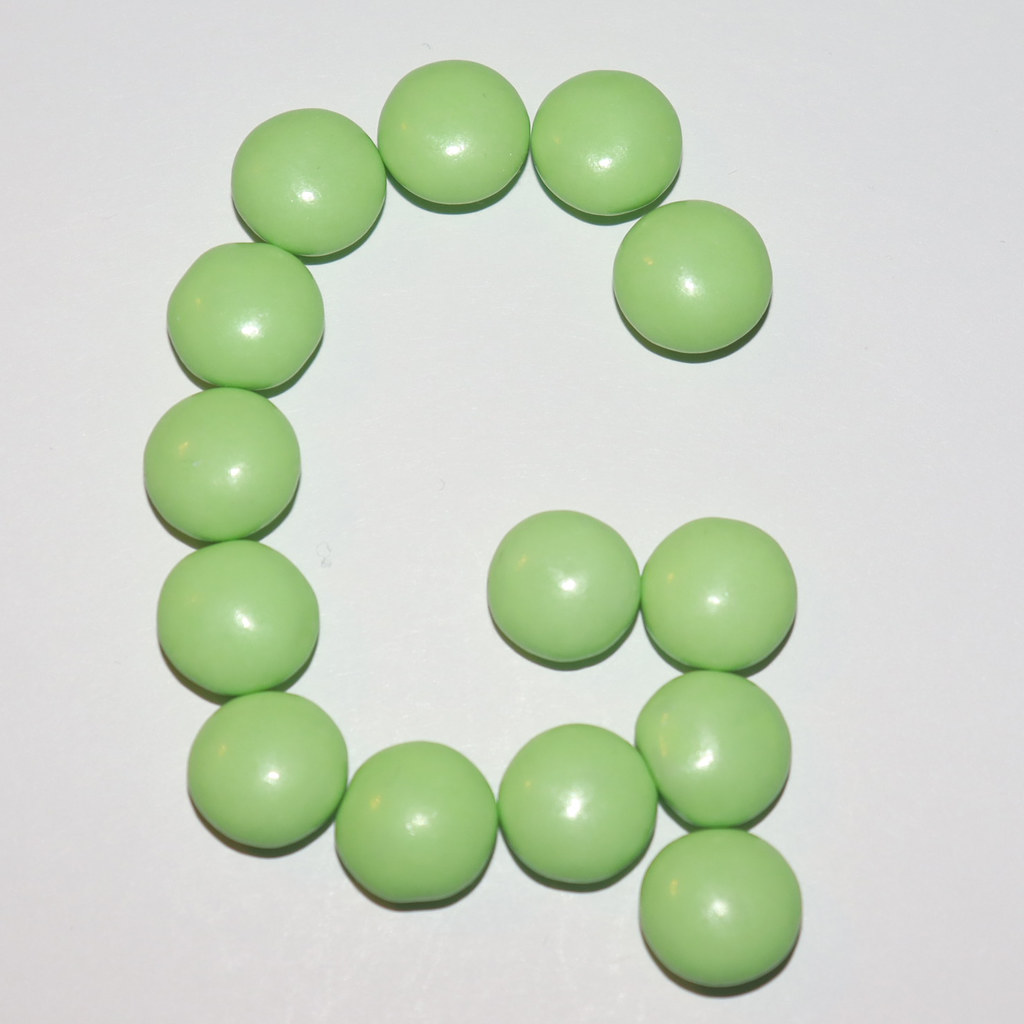The image depicts 14 light lime green, slightly irregularly shaped round candies or game pieces arranged meticulously on a plain white background to form a capital letter G. Each piece, which has a subtle shiny sheen, exhibits a reflection of light, likely from a camera flash or an overhead light source.